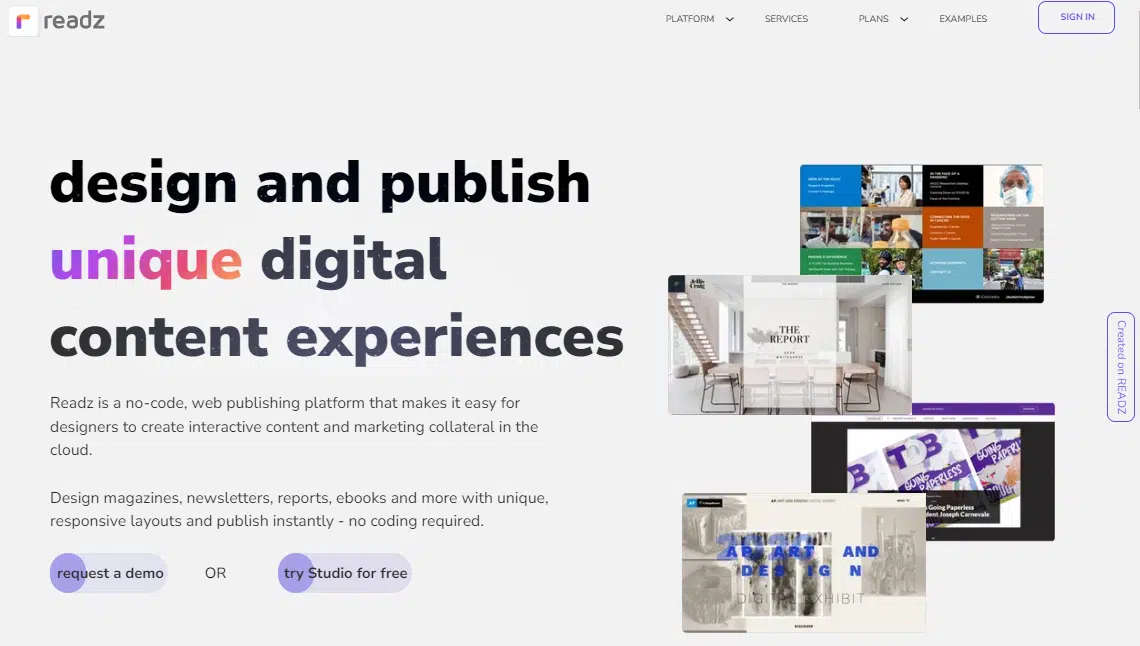This webpage features the web publishing platform "Reads" (stylized as READZ), distinguished by its logo of a right-angled, lowercase "r" in vibrant colors. The main slogan, "Design and Publish Unique," is prominently displayed in shades of blue and purple, while the supporting text appears in grey and black. The comprehensive message reads: "Design and Publish Unique Digital Content Experiences."

Reads is a no-code web publishing platform tailored for designers, enabling the creation of interactive content and marketing materials directly in the cloud. This includes the design of magazines, newsletters, reports, ebooks, and more, all with unique responsive layouts that can be published instantly — no coding required.

A call-to-action button beneath this message offers users the options to "Request a Demo" or "Try Studio for Free." To the right of this text, several images showcase examples of the types of publications created using the platform. These include a multi-sectional layout and full-page designs, illustrating the diverse and dynamic content that Reads can help designers produce.